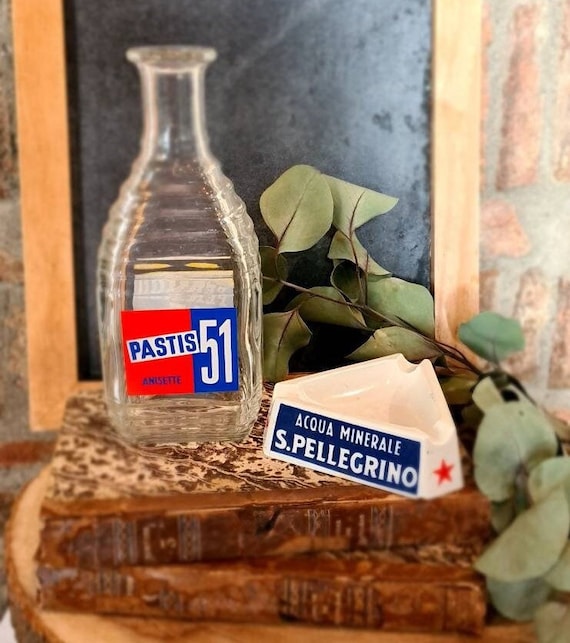On an end table, there are two worn, brown-spined books stacked on top of each other. Resting on these books is a translucent glass bottle with ribbed sides and a narrow neck. The label on the bottle features a red background on the left side and a blue background on the right, with "Pastis" written in blue and "51" in white. Next to the bottle, there's a white, triangular ashtray adorned with dark blue and white text that says "ACQUA MINERALE S. Pellegrino," alongside a distinctive red star. Draped over the lower right quadrant of the setup is a green, leafy vine, adding a touch of nature. In the background, a framed blackboard, devoid of any writing, hangs on the wall behind the table.